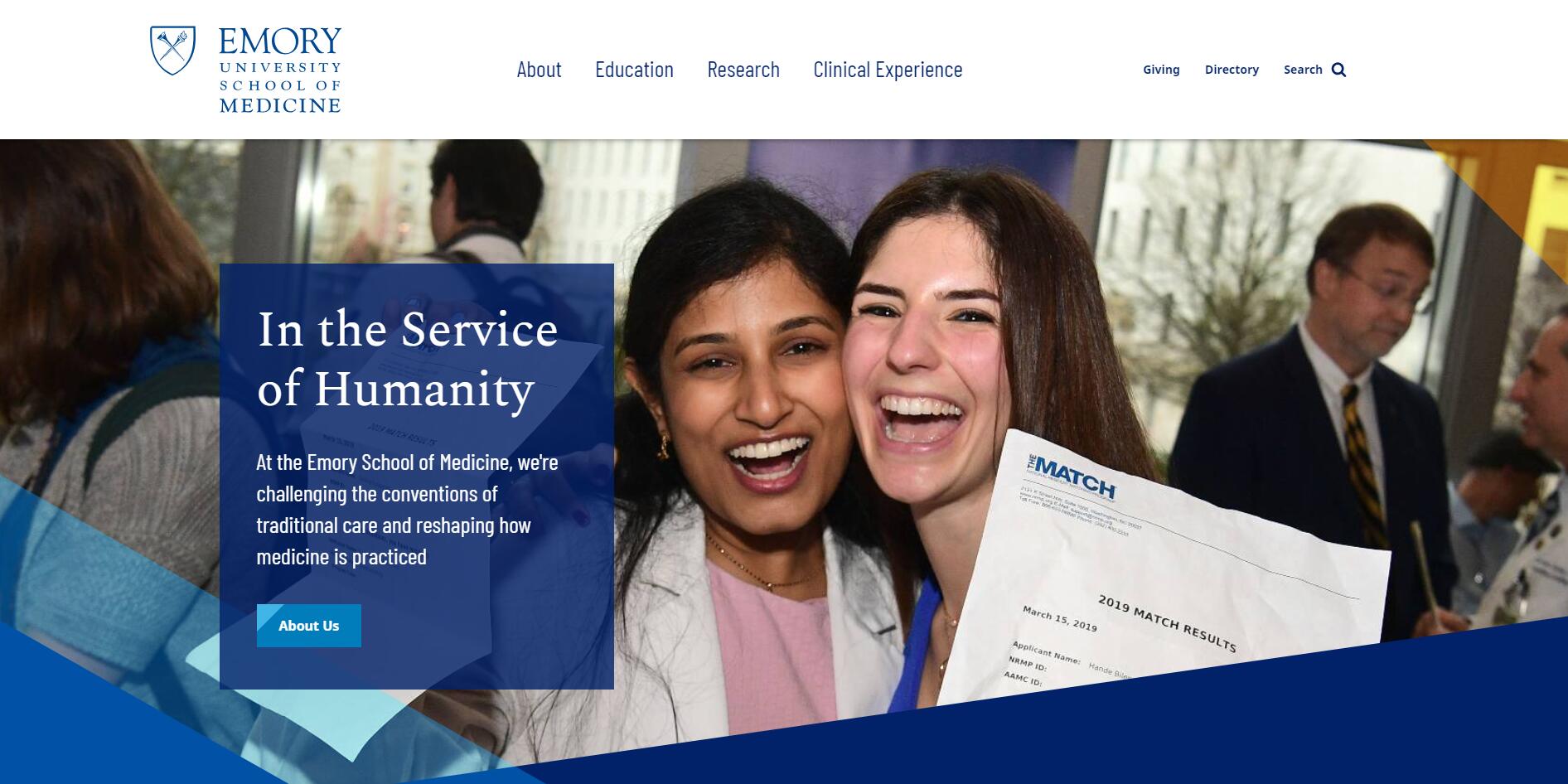The image depicts the homepage of the Emory University School of Medicine's website. Prominently displayed in the top left corner is the name of the institution accompanied by a blue shield-like icon. Inside the shield, two syringe-like shapes form an 'X'. Centered at the top of the page are four navigational categories labeled "About," "Education," "Research," and "Clinical Experience." To the far right, there are three additional links labeled "Directory," "Search," and next to a small blue magnifying glass icon, "Give."

In the middle section of the webpage, a text box on the left contains an inspirational message: "In the service of humanity. At the Emory School of Medicine, we're challenging the conventions of traditional care and reshaping how medicine is practiced." Below this, there is a smaller box with the text "About Us." The background image features a diverse group of people, with two women prominently positioned in the foreground. The woman on the right has a fair complexion and brown hair, while the woman on the left has a darker skin tone and black hair, and is dressed in a white medical coat.